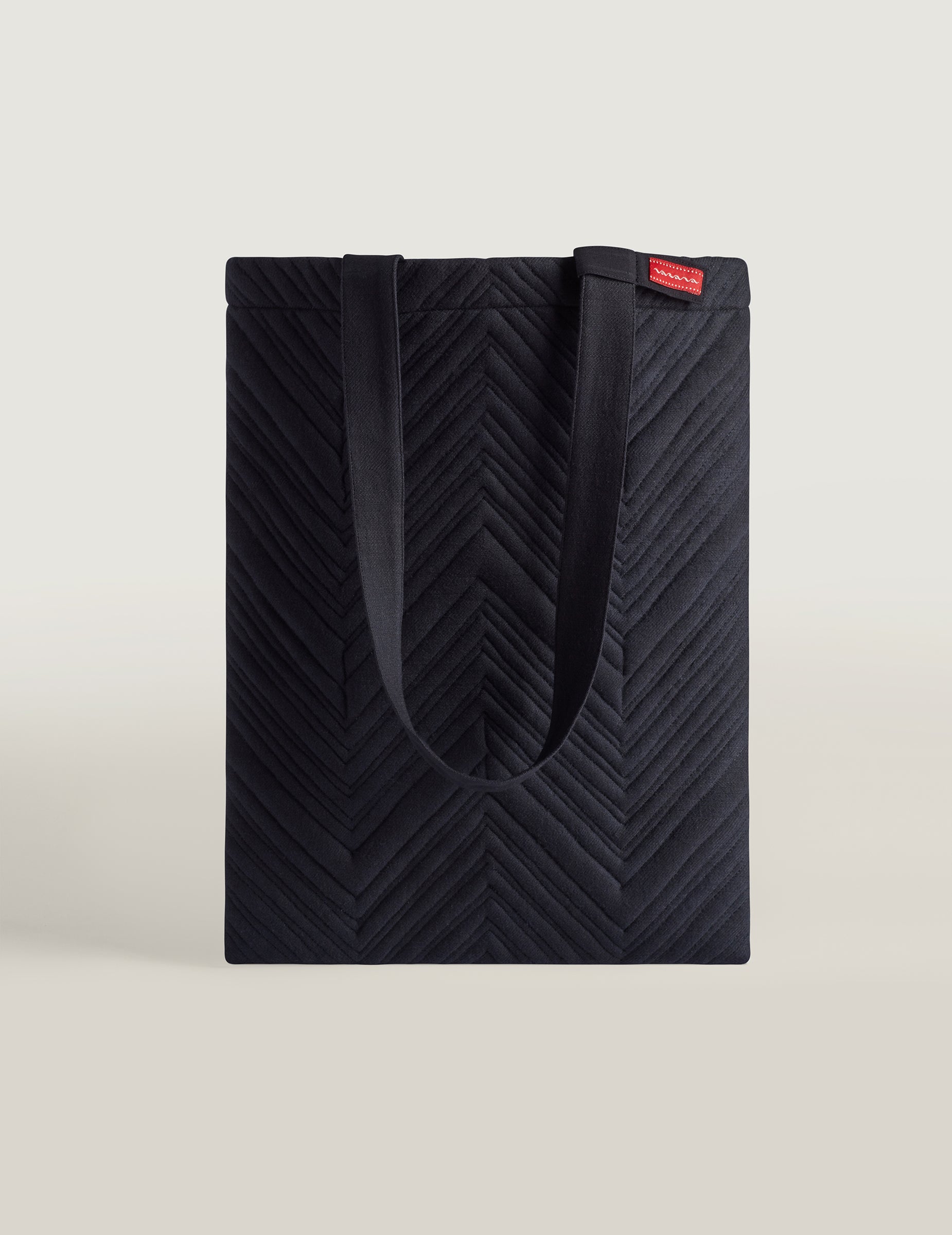The advertisement photo features a vertically oriented black handbag or tote bag, positioned on a white surface against a white background. The bag, designed to be carried by hand or on the arm, is primarily composed of black fabric with a distinctive chevron pattern that extends from the top to the bottom. Notable details include a black handle and a prominent red tag with white letters, located near the top right-hand side of the bag. The small red tag, possibly adorned with gold designs or writing, adds a subtle yet striking contrast to the black fabric. The bag's shape resembles a rectangle, suggesting versatility for carrying items such as books, laptops, or essentials, although its exact dimensions remain unspecified.